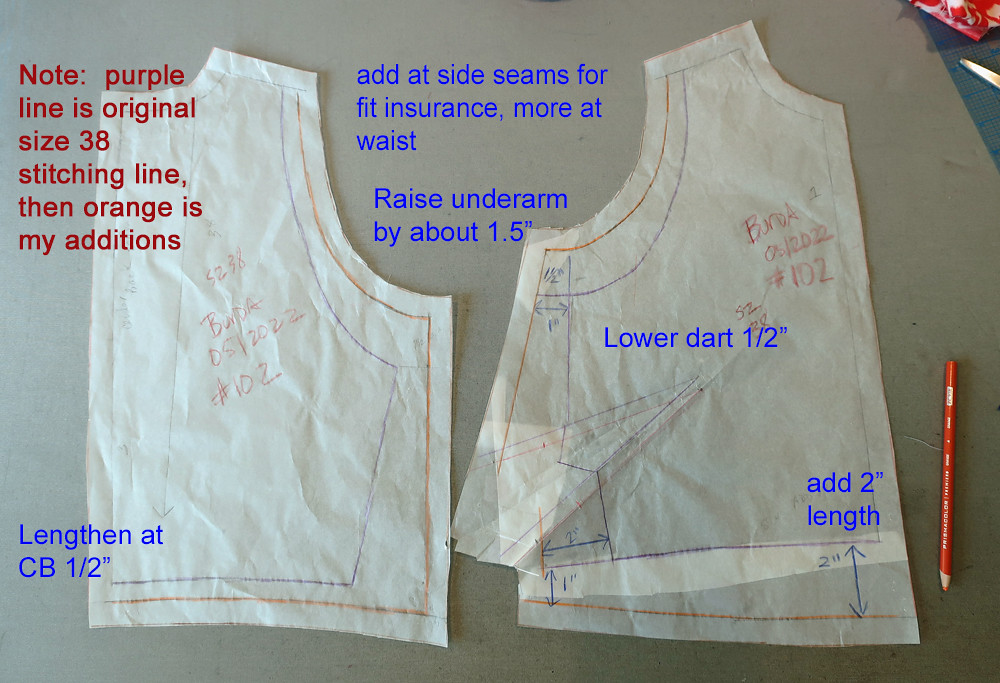This detailed photograph captures a pattern-making workspace set against an off-white or gray table. At the center, pieces of paper with various stitching lines and instructional markings dominate the scene, accompanied by a pencil placed to the right. The papers feature handwritten notes and lines in multiple colors, including gray, red, white, blue, pink, silver, and orange. Prominent text includes detailed directions for adjusting and customizing a clothing pattern: “Lower dart half inch,” “Add 2 inch to the length,” “Lengthen at CB half inch,” “Raise underarm by about 1.5 inches,” and “Add at side seams for fit insurance, more at waist.” Blue text highlights additional adjustments for fitting. The setting suggests an indoor environment, potentially an arts and crafts room, dedicated to the meticulous craft of garment creation.